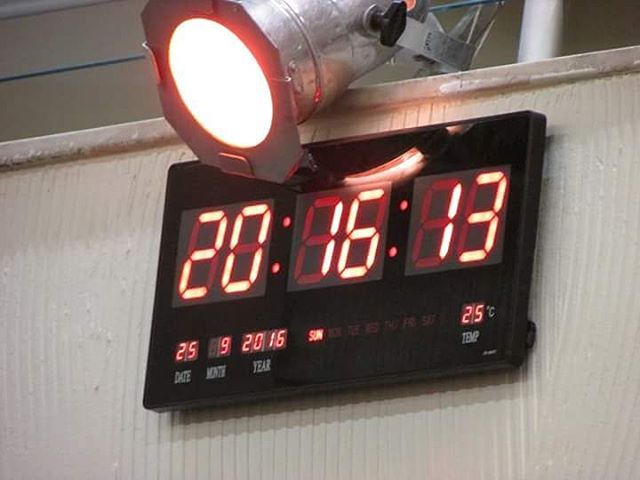This image features an industrial-style digital clock, prominently displayed on a textured wall, possibly within an events venue or sports rink. The clock's face is black, contrasting with the brightly lit digital readouts. Illuminated by an overhead industrial light, the clock provides a range of data: it shows the time as 20:16:13, the date as September 25, 2016 (a Sunday), and the temperature as 25 degrees Celsius, suggesting it might be intended for an international or non-American audience. The background includes a metal railing at the top, with visible metal poles and cords, adding to the utilitarian aesthetic of the setting.